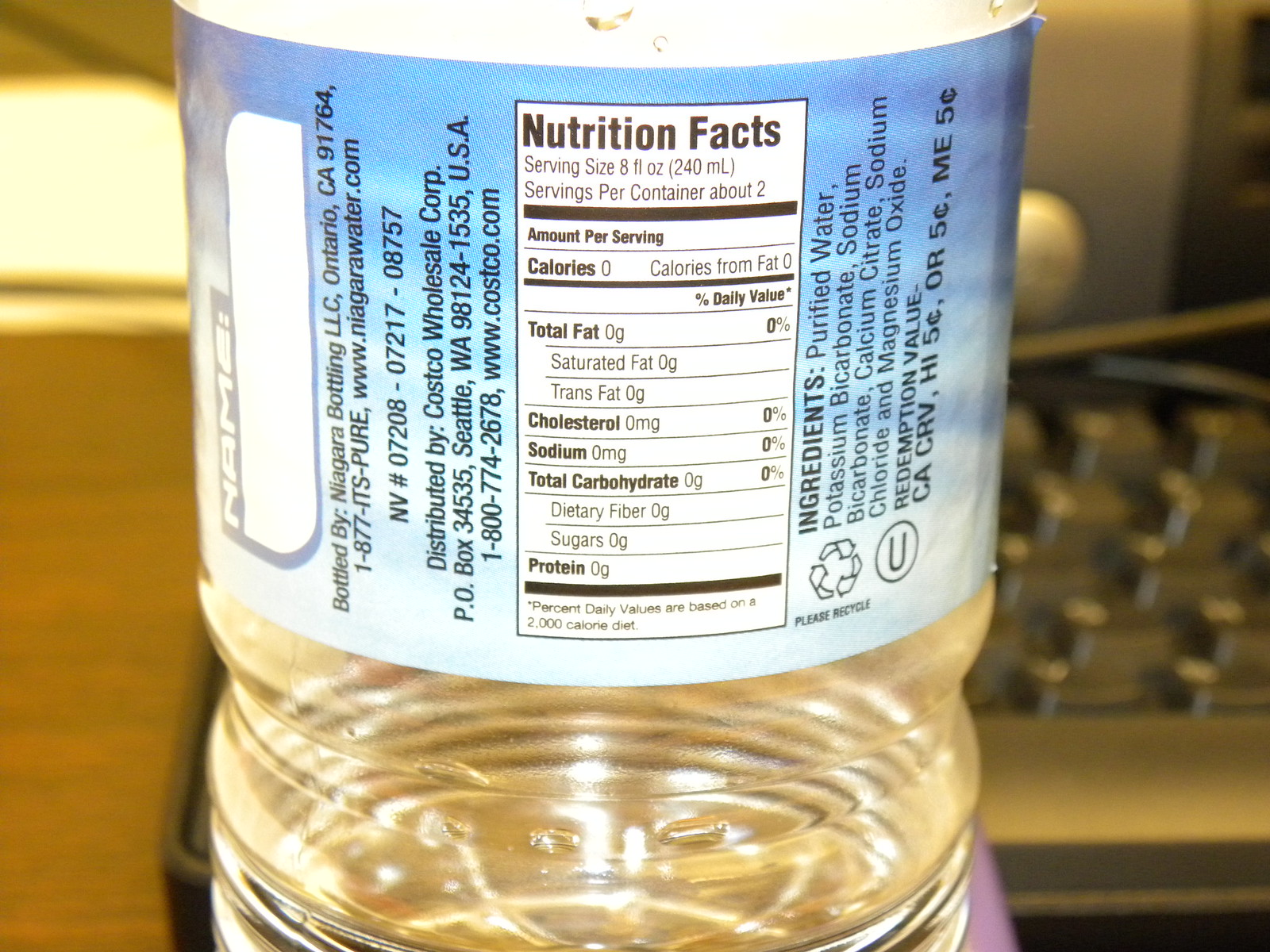This close-up photograph captures a detailed view of the back label of a plastic water bottle. The focal point is a designated section for writing one's name. The label provides a variety of information, including the bottling location, which lists Niagara in Ontario, California. Additionally, it features the company's website, customer service phone number, barcode, and other product-related numerals. The mention of Costco as the distributor is prominent, along with their address, phone number, and website specifics. Centrally located on the label is the nutritional facts chart, highlighting the absence of calories and sodium. To the right, the ingredients are listed, mainly purified water, along with magnesium, sodium, and chloride. The label also displays logos such as the recycling symbol and information regarding recycling costs. The background reveals the bottle is placed behind a computer table, where parts of a keyboard and computer are visible.